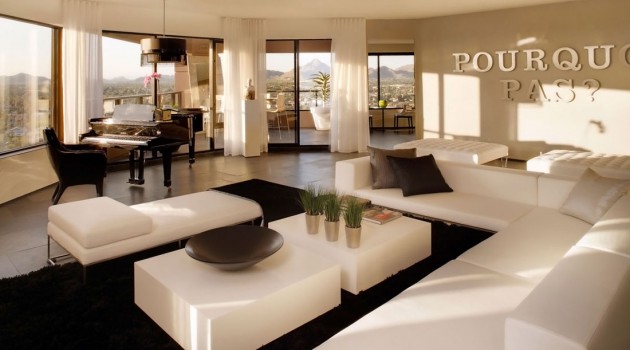The image showcases an opulent high-rise penthouse living room featuring four expansive floor-to-ceiling windows along the back left wall that flood the space with natural light and offer views of neighboring buildings, including an office building and mountain scenery. The centerpiece is an open baby grand piano with exposed keys, accompanied by a standard chair. The polished hardwood floor supports an elegant array of cream-colored leather furniture, including a large L-shaped sectional sofa decked with three 18-inch square throw pillows in brown, black, and a lighter cream shade.

A black rug defines the seating area, accentuated by two low, square coffee tables. One table holds a distinctive black bowl shaped like a wok, while the other displays three identical potted plants alongside a magazine. Adjacent to the sectional is a white chaise lounge, also resembling a daybed, resting on the same black rug.

The room's decor is complemented by white curtains drawn to the sides of the tallest window, and the reflections of sunlight dance across the spaces, adding warmth and emphasizing the luxurious feel. On a sunlit wall, partially obscured capitalized letters spell out "P O U R Q U E P A S," adding a mysterious and artistic touch to the sophisticated setting.